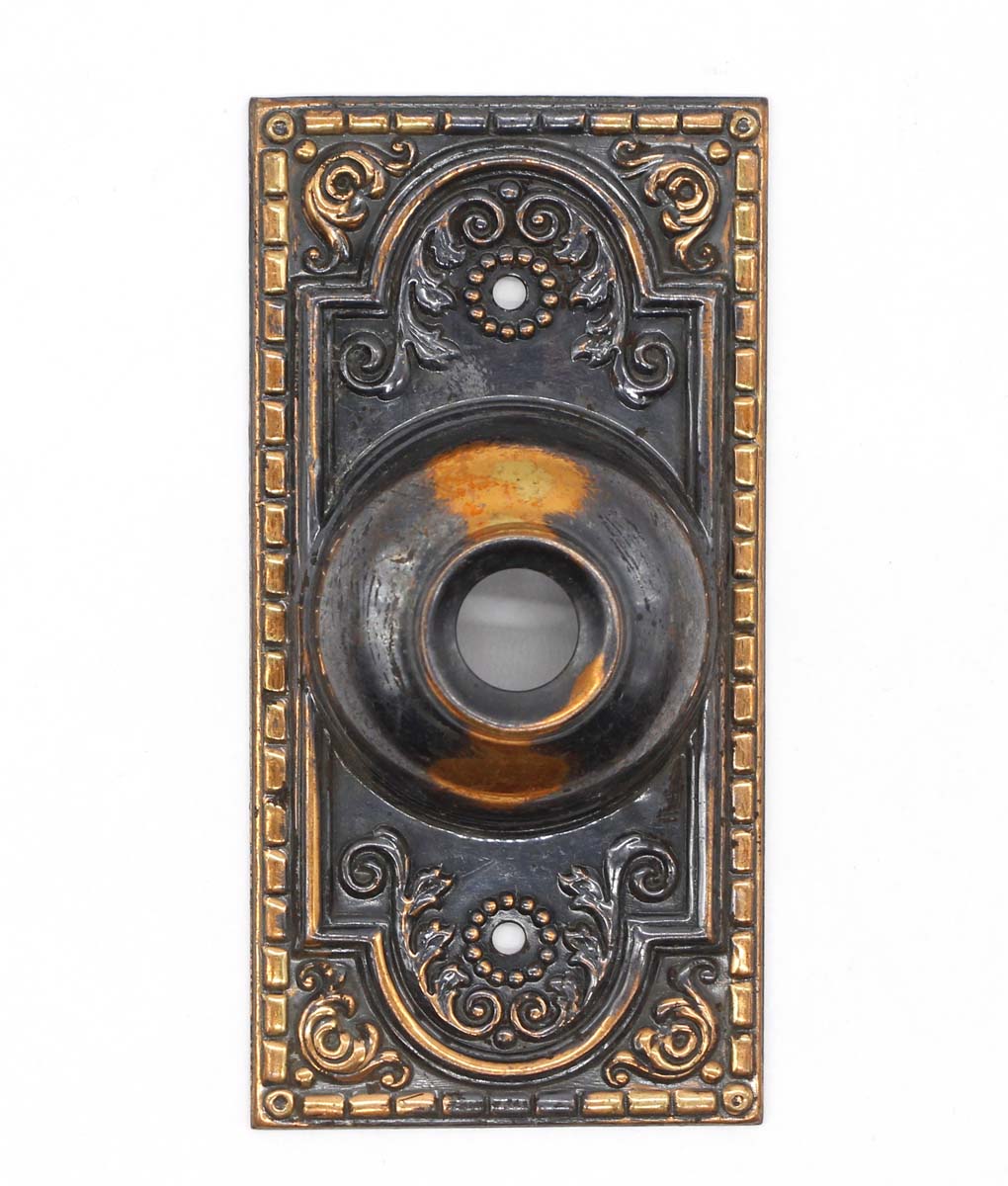This image depicts an ornate and decorative doorpiece likely serving as either a doorbell or doorknob casing. The rectangular plate is crafted from heavy metal exhibiting a rich interplay of black and gold tones, possibly due to aging and wear. Around the edges, small decorative rectangles are meticulously lined, with floral-like swirls embellishing each of the four corners. At the center lies a prominent black circle with a white spot, suggestive of a doorbell to be pressed. Complementing this design are two smaller white circles, positioned above and below the central circle, and each outlined with delicate gold dots. The intricate design also includes swirling lines and rounded squares interwoven with dot patterns, enhancing its luxurious and antique aesthetic.